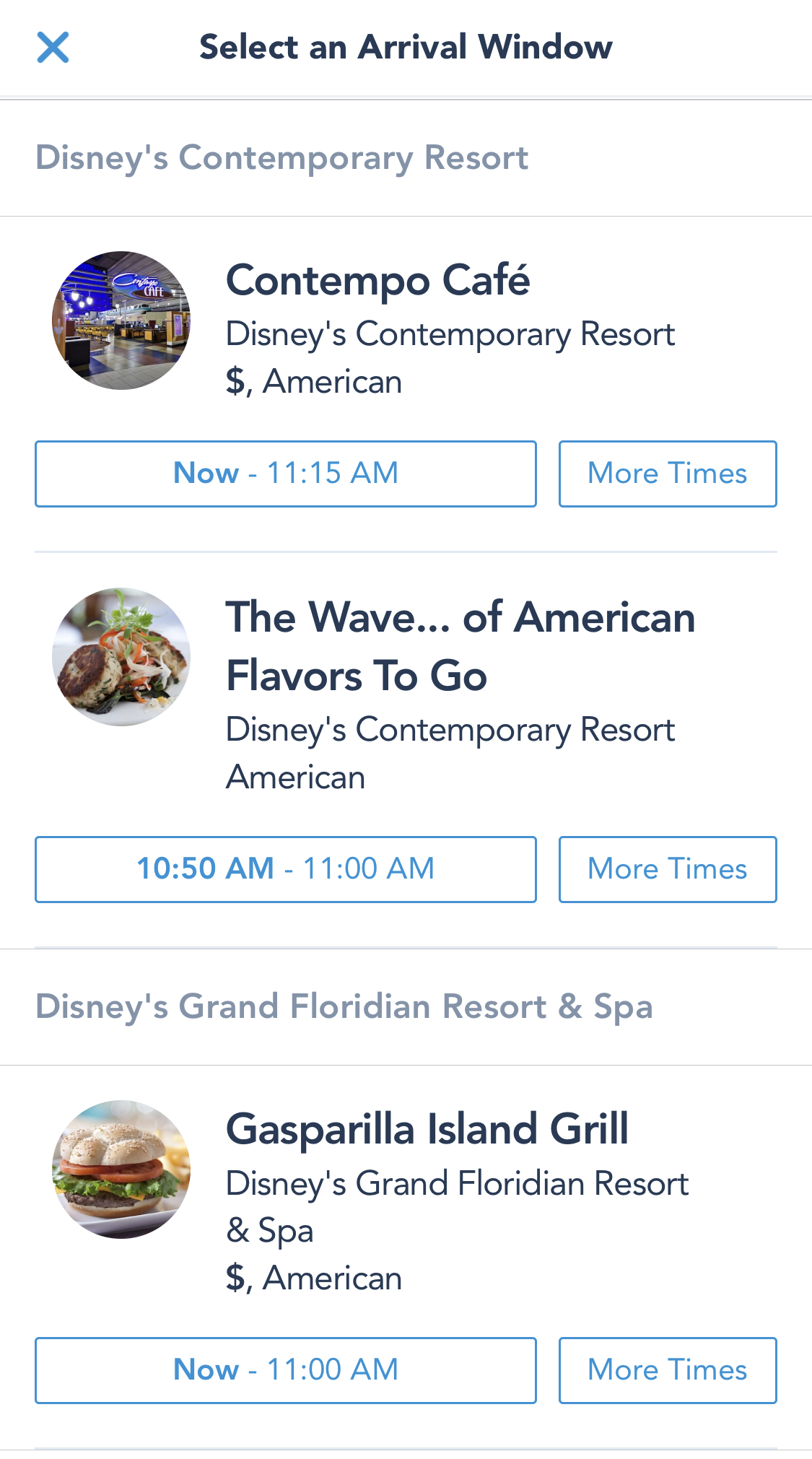The image displays a booking screen for selecting an arrival window at one of three restaurants within Disney's Contemporary Resort. The top section of the screen prompts the user to "Select an Arrival Window." The available options include:

1. **Contempo Cafe, Disney's Contemporary Resort** – Arrival window from now until 11:15 a.m.
2. **The Wave of American Flavors To Go, Disney's Contemporary Resort** – Arrival window from 10:50 a.m. to 11:00 a.m.
3. **Gasparilla Island Grill, Disney's Grand Floridian Resort and Bar** – Arrival window from now until 11:00 a.m.

Each restaurant option is accompanied by an image showcasing the type of food available at that venue, providing a visual representation of the dining experience. The purpose of the menu is for users to book a reservation by selecting a preferred arrival time at one of the three restaurant options.